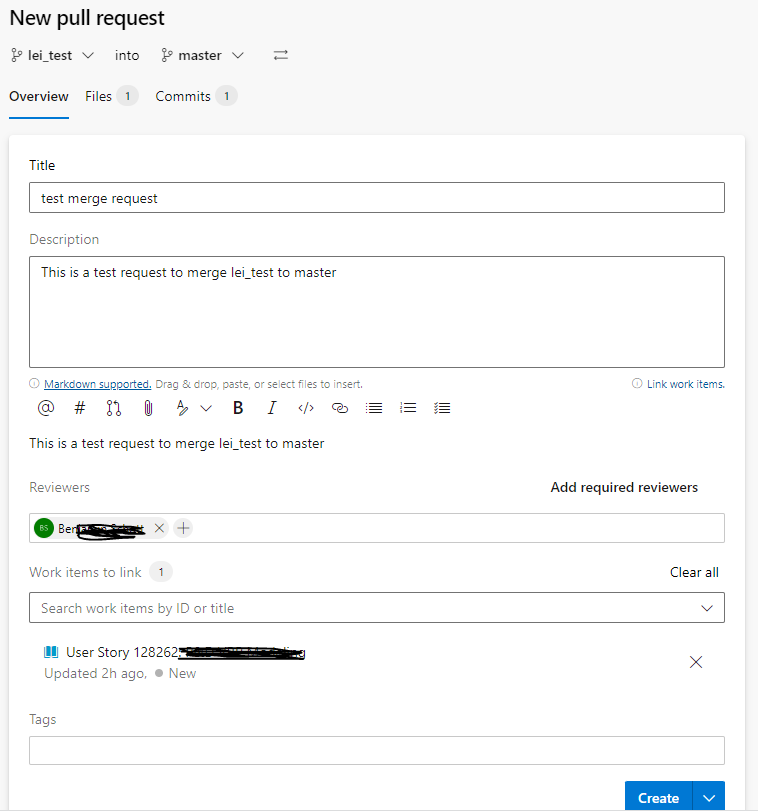This image is a screenshot taken from a computer interface, showing the creation of a new pull request. The background is white with black text, prominently displaying "New Pull Request" at the top. In the upper left-hand corner, there's a drop-down menu labeled "LEI_test." Adjacent to it, another drop-down menu is labeled "into master." 

Below these options, filters are available, with the "Overview" tab currently selected, indicated by a blue underline. To the right side of this section, two tabs show: "Files" and "Commits," each accompanied by a circular icon containing the number "1."

The screenshot then focuses on the title and description sections for the pull request. The title field contains the text "Test Merge Request." In the description area, it reads, "This is a test request to merge LEI_test to master." Additionally, the description box offers a blue hyperlink for "Markdown supported." Below this, there are instructions stating, "Drag and drop, paste, or select files to insert," accompanied by another hyperlink labeled "link work items."

Further interface options are shown for text formatting, including buttons for bold, italic, an "@" symbol, hashtag, and a paperclip icon, likely for attachments. At the bottom of the image, the "Reviewers" section is visible, though no specific reviewers are listed or highlighted.

Overall, this is a detailed depiction of the pull request creation interface, highlighting various fields, options, and functionalities available to the user.